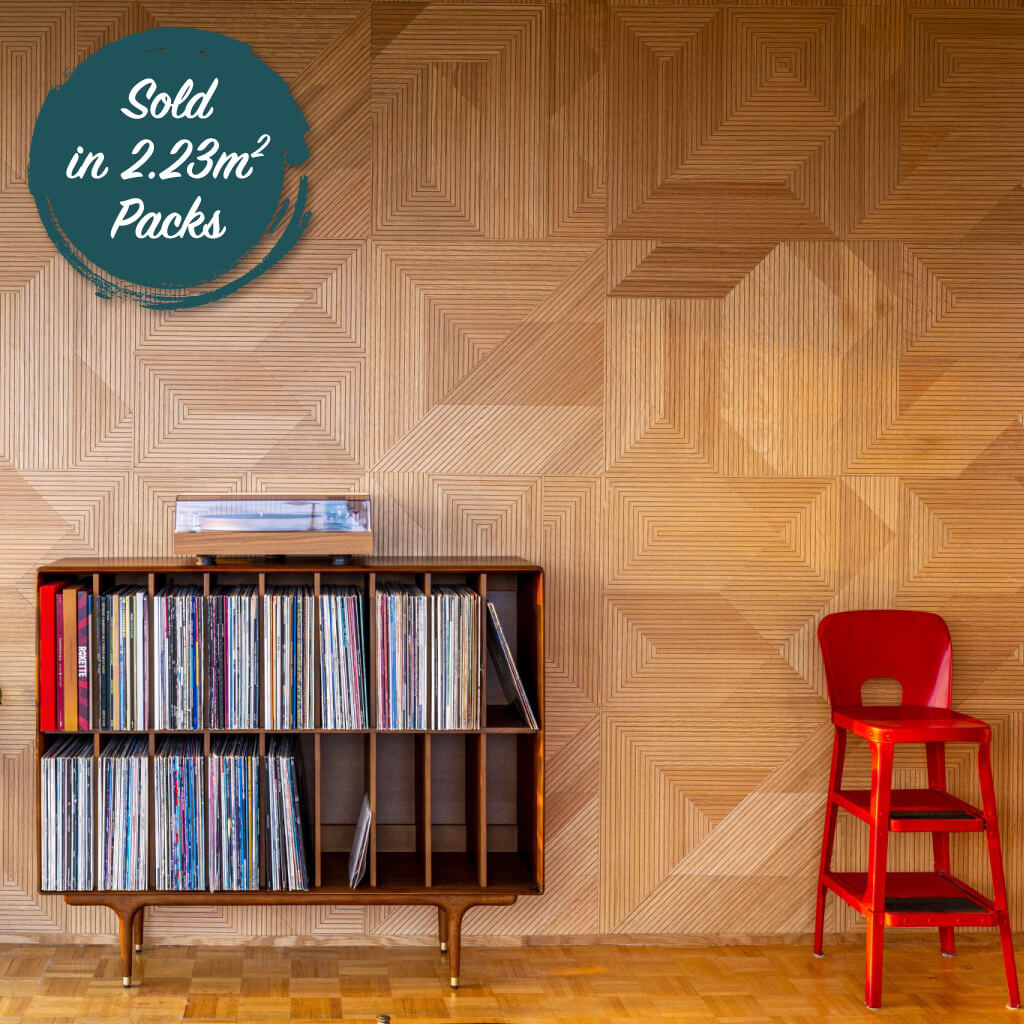The image portrays a vintage room setting, dominated by a tan, textured paneled wall adorned with geometric designs. The floor complements the wall with its parquet wooden tile pattern. Central to the scene is a wooden console table designed to store vinyl records, divided into two shelves with nine slots each. The upper shelf is nearly filled with a colorful collection of record albums, while the lower shelf holds fewer items. Atop the console rests a turntable within a plastic cover. To the right of the console, and accentuating the retro vibe, is a bright red metal step stool with a short back and two shelves underneath, resembling a 1950s style. Completing the advertisement-like appearance is a green circle in the upper left corner with the inscription, "Sold in 2.23 M squared packs."